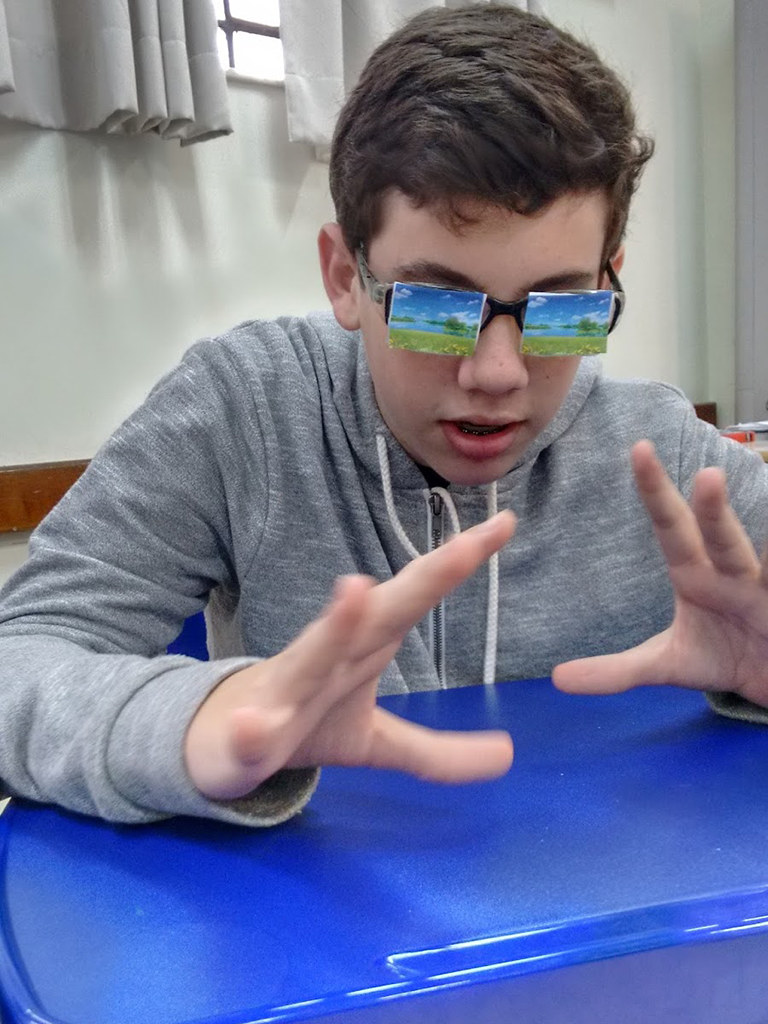This color photograph depicts a young Caucasian boy with short black hair, wearing a gray hoodie with white drawstrings. Seated in front of a desk with a royal blue plastic surface, he holds his hands out in front of him, almost as if making a square shape with his fingertips. His glasses, adorned with high-resolution images of an outdoor scene featuring a blue sky with clouds, water, trees, and green grass, obscure his eyes. The backdrop includes a gray wall with a window dressed in short gray curtains and an orange-brown skirting board at the base. The boy appears to be looking down towards his hands, adding depth to the composition.